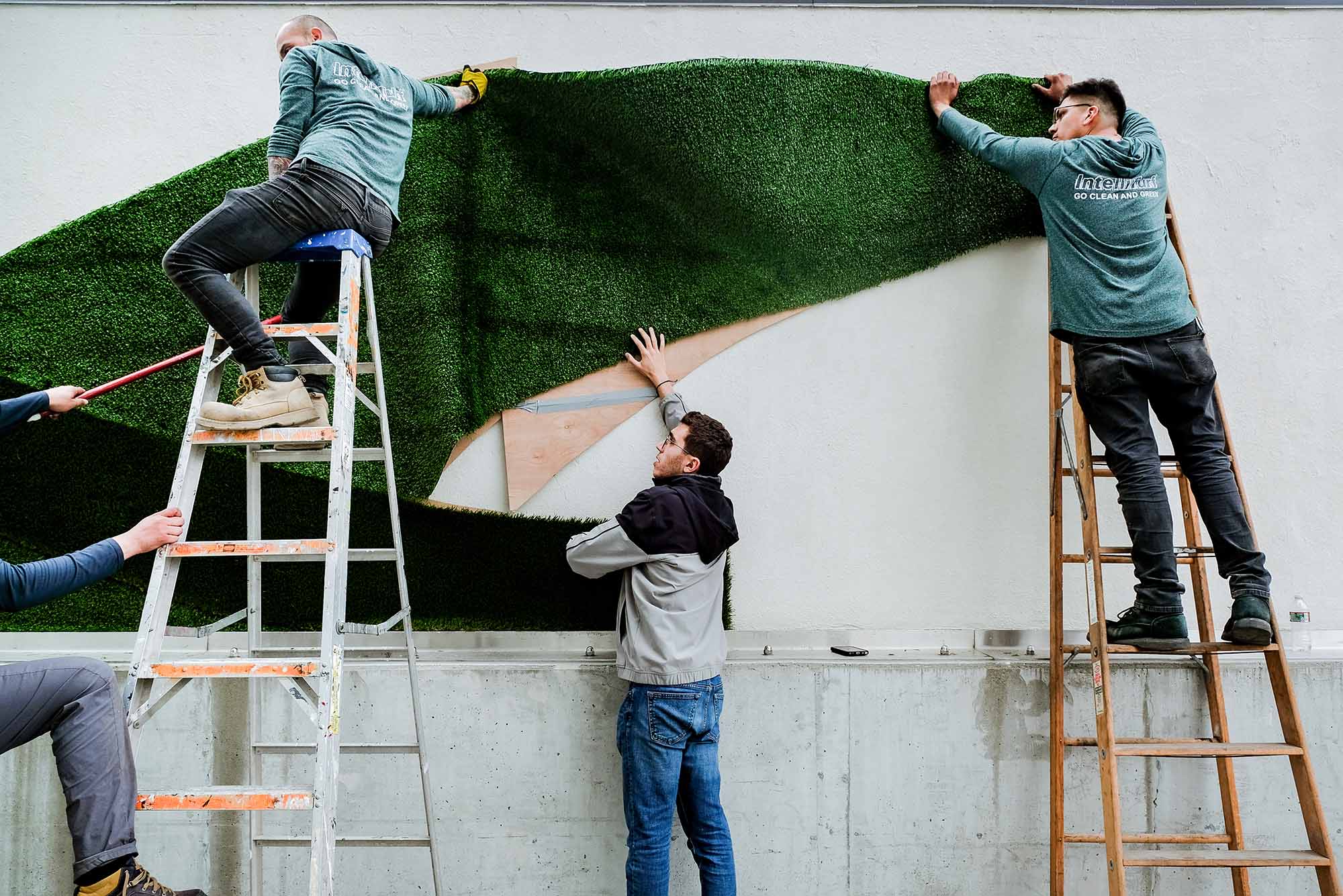In the image, four men are meticulously working together to mount a curved section of green astroturf onto a light gray concrete wall. Two of the men are seated atop step ladders, one on a metal ladder to the left and another on a wooden ladder to the right. Both are holding and positioning the astroturf while wearing jeans and matching blue shirts. The man on the metal ladder wears a turquoise sweatshirt and looks towards a man partially cut off by the left edge of the photo, identifiable only by his jeans and long blue sleeves as he stabilizes the ladder. In the center, a man in a white jacket and jeans stands on the ground, holding the bottom edge of the astroturf, aligning it carefully. A mounting bracket is visible on the wall, and one of the men brushes the astroturf's surface gently. The setting appears to involve some form of stage or screen set-up, as indicated by a phone resting on a nearby platform. The unified effort showcases the detailed and coordinated task of positioning the astroturf accurately on the wall.